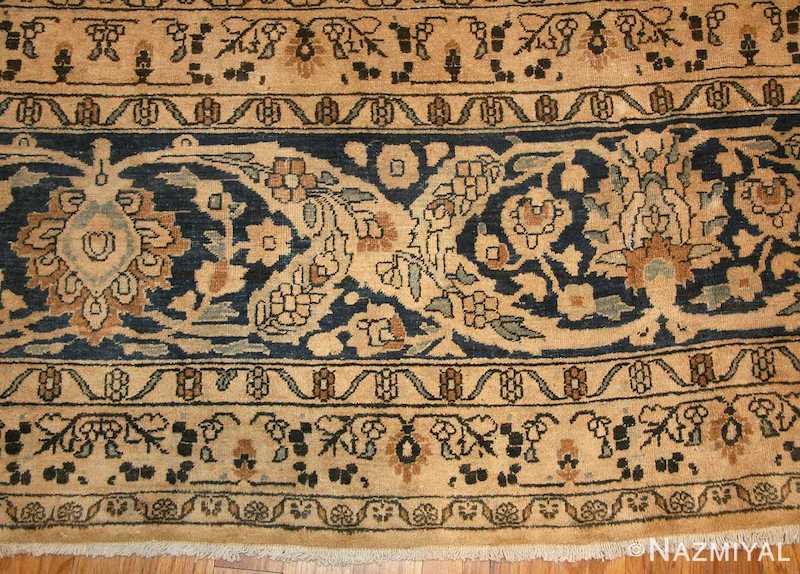This image captures a beautifully detailed Persian-style rug displayed on a polished wooden floor. The rug features a rich tapestry of intricate floral designs, meticulously woven into the fabric. The main body of the rug is a light cream or tan color, accented with various shades of blue, dark blue, and touches of brownish-yellow, orange, and red.

The pattern is organized into horizontal rows, each showcasing different motifs. At the top, there is a narrow border adorned with flowers and vine-like designs. Below this, a wider section depicts a lavish display of flowers and leaves, all set against a dark blue background. This primary section is flanked by narrower rows of smaller, daisy-like flowers and intricate patterns, creating a mirror image effect above and below the wide central area.

The rug is finished with a delicate white fringe along the bottom edge, beneath which a small strip of the wooden floor is visible. In the lower right corner of the photograph, the word "Nazmayal" (N-A-Z-M-I-Y-A-L) is prominently displayed, likely indicating the maker or copyright holder of the image. This exquisite textile, possibly an heirloom-quality floor rug, showcases traditional Persian floral iconography with a sense of timeless elegance.